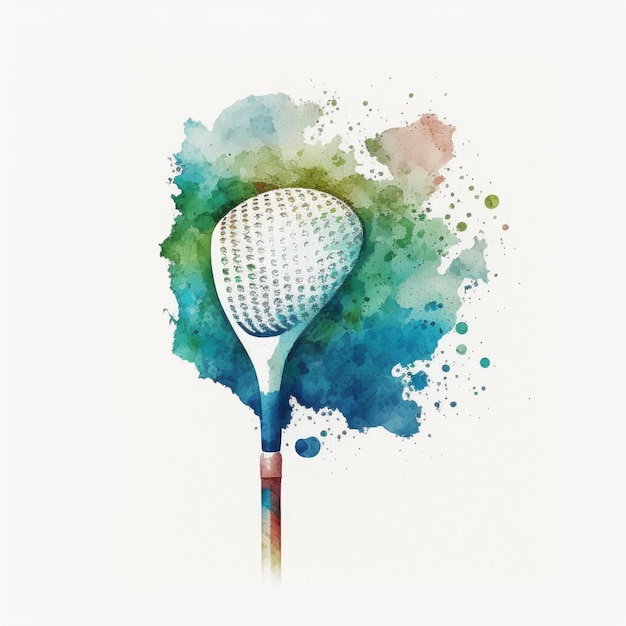This horizontal-rectangular image is an abstract, watercolor-like painting centered around a vintage wooden-shafted golf club. The golf club’s head, positioned slightly off-center to the left, features a distressed metal appearance, characterized by numerous small polka dots that add texture to its surface. A distorted golf ball, appearing squished, is superimposed onto the club head. The wooden shaft transitions from a bluish color where it joins the club head, and fades into pinks and maroons as it extends upwards. The background is a vibrant, spontaneous splash of color, with deep blues at the bottom gradating into greens and hints of yellow-green, topped off with pink accents. The watercolor paint, applied haphazardly, creates a splotchy effect with scattered dots around the composition, contributing to the painting’s dynamic and textured appearance. The entire artwork is set against a cream-colored paper, enhancing the watercolor's fluid and translucent quality.